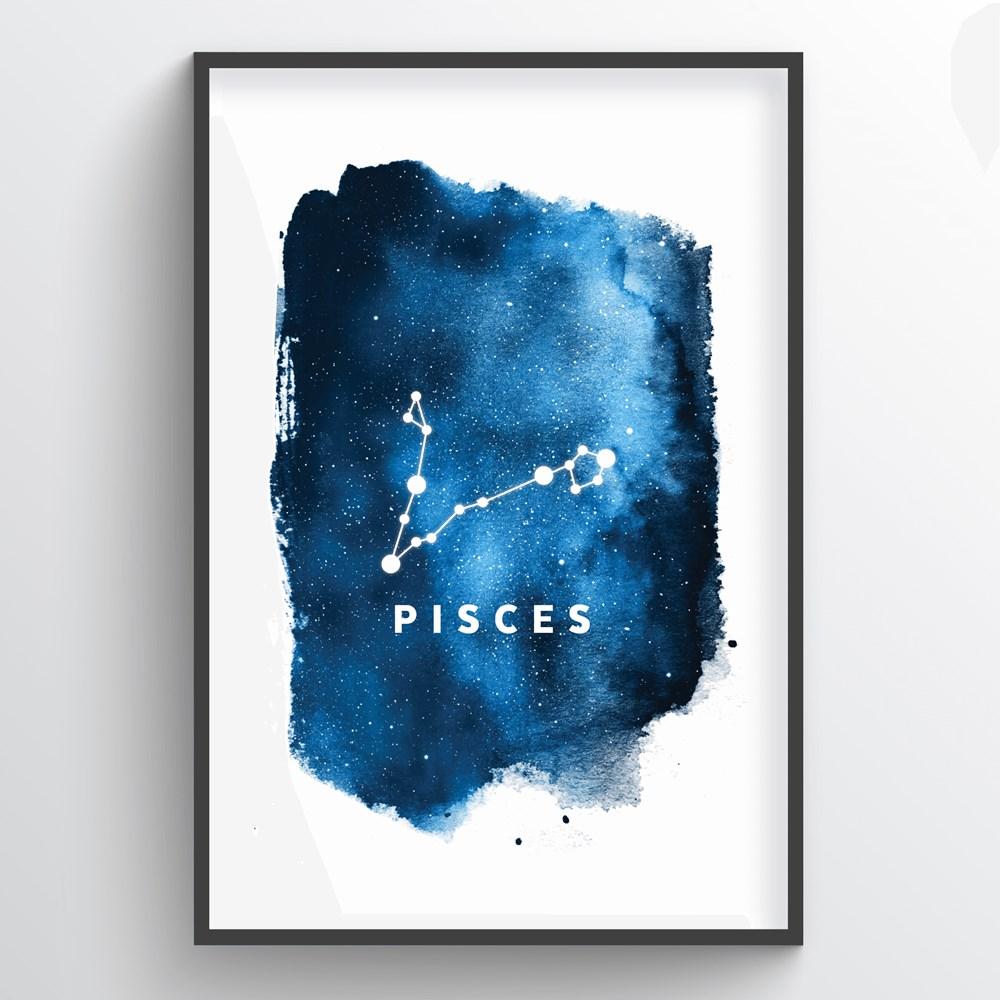This indoor photograph showcases a framed illustration of the Pisces constellation, hung on a white wall. The picture is encased in a thin, classic black frame, potentially wooden, with possible shadowing that suggests an inset or glass cover. Presented in a vertical, portrait orientation, the artwork within features a watercolor or print depiction of a star field. The background transitions from a deep blue to lighter blue hues, with raw, jagged edges and occasional splatter marks extending beyond the painted area. In the center of the piece, the constellation Pisces is illustrated with major stars represented by larger white dots and minor stars by smaller ones, all interconnected by straight white lines. The name "PISCES" is prominently displayed across the middle in clean, modern capital letters with wide kerning. The image conveys a sense of depth and celestial beauty, enhanced by the white lettering and absence of extraneous markings. The background of the painting surrounding the watercolor remains white, providing a stark contrast that highlights the constellation's design.